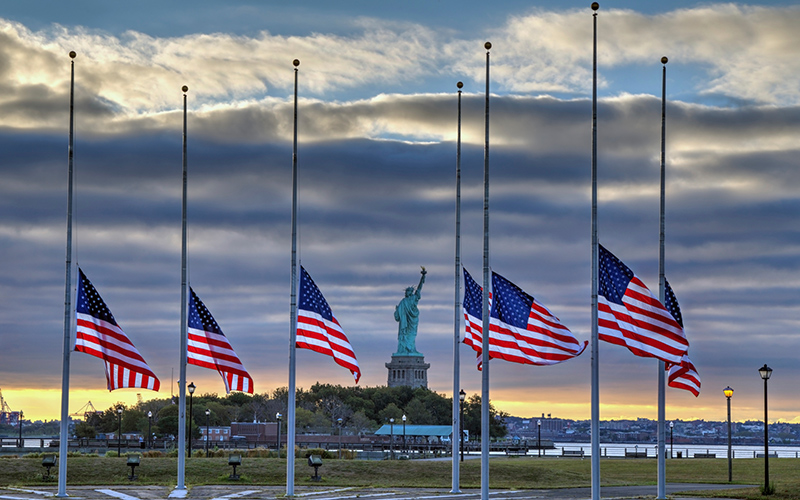The image depicts a poignant scene on Liberty Island in New York City, with the iconic Statue of Liberty standing tall in the background amidst lush vegetation. Seven American flags are prominently displayed, each at half-mast, likely commemorating a recent tragedy. These flags are arranged in a circle, with several benches visible behind them, facing the tranquil waters of New York Bay. The sky, adorned with clouds, suggests either sunrise or sunset, casting a serene yet somber backdrop to the memorial. Unlit lights are positioned to illuminate the flags at night, completing the reflective atmosphere of this revered site.